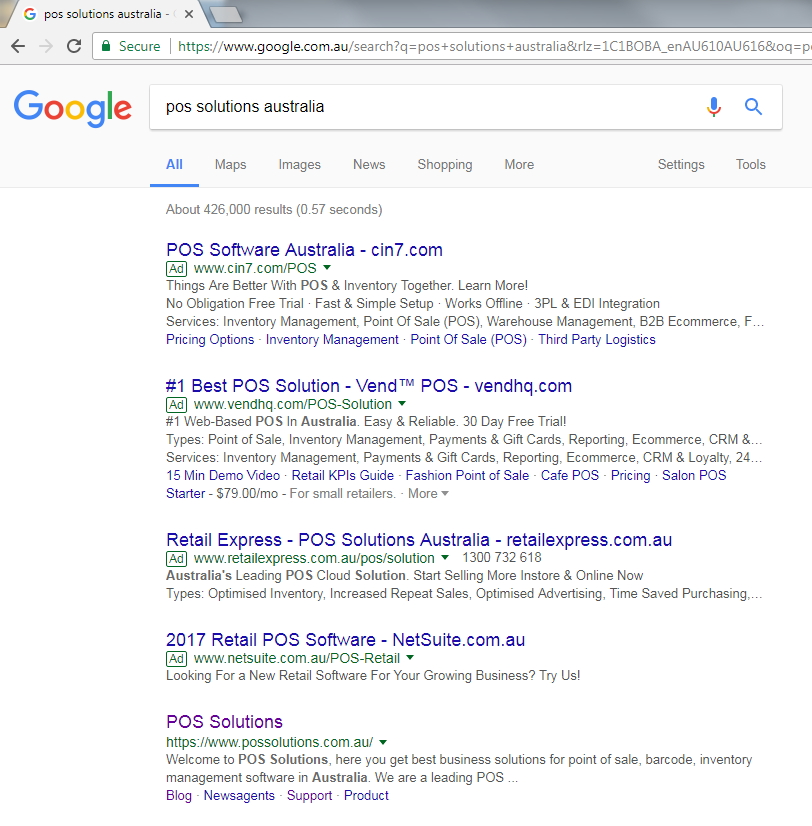This screenshot captures a Google Chrome browser displaying search results for "POS Solutions Australia." The browser tab is labeled "POS Solutions Australia," and the familiar Google header is present, featuring the Google logo and a search box pre-filled with "POS Solutions Australia." Beneath the search box are various navigation tabs: All, Maps, Images, News, Shopping, More, along with Settings, and Tools options. 

The search yields approximately 426,000 results, with the top five or six prominently featured. The first four results are designated as advertisements and indicated by an "Ad" label next to their URLs. These results include:
1. "POS Australia" from SIN7.com.
2. "Number One Best POS Solutions" from VandPOS at VandHQ.com.
3. "Retail Express POS Solutions Australia" from RetailExpress.com.au.
4. "2017 Retail POS Software" from NetSuite.com.au.

The fifth result is an organic listing without the "Ad" label:
5. "POS Solutions" from POSSolutions.com.au.

Each search result features a brief description, a green URL, and, where applicable, the "Ad" designation.